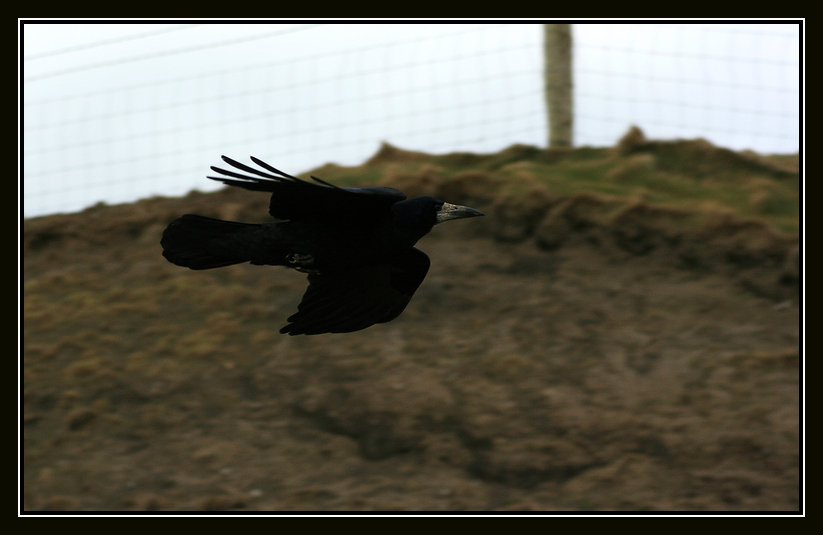This image captures a dynamic moment of a black bird, likely a crow, in mid-flight, soaring from left to right against a blurred backdrop. The crow is entirely black, with striking details such as a grayish-black beak and black feathers that fan out in a spread-finger manner on its wings, while its closed tail feathers form a fan shape. The bird, centered in the photograph, appears to be moving swiftly through the air, evident from its streamlined and aerodynamic positioning. The background, though out of focus to emphasize the crow, features a network of crisscrossing wire fences arranged in a grid pattern, anchored by a prominent wooden post in the center. The scene suggests a hilly area with sparse vegetation or mounds of dirt, under a sky that hints at diffuse daylight, possibly on a foggy or cloudy day. The simplicity and minimalism of the surrounding elements bring the viewer’s attention squarely on the bird's elegant and fast flight.